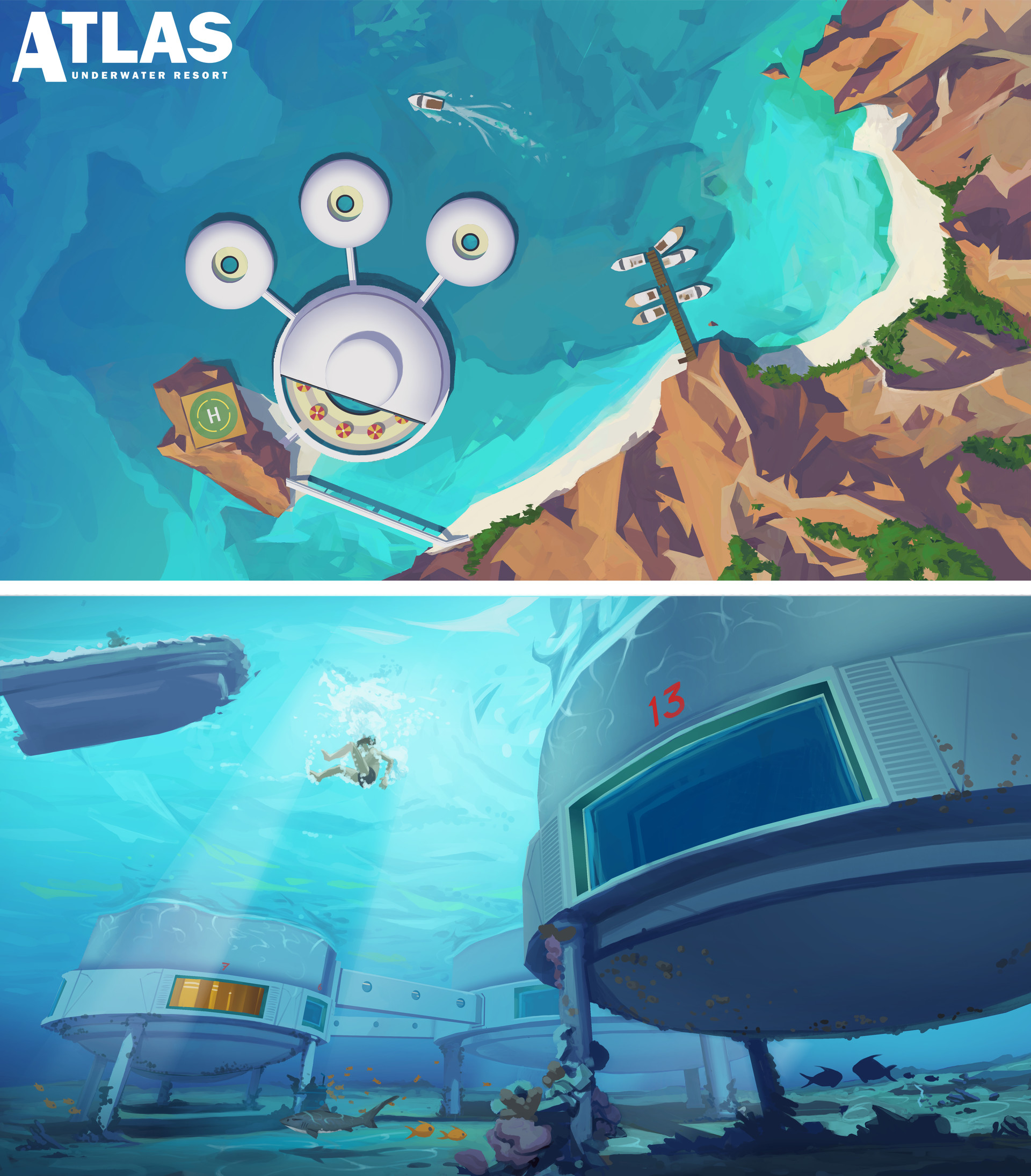The image is a digitally created advertisement divided into two sections, one on top of the other.

In the top section, large capital letters spell out "Atlas" in white text, followed by "Underwater Resort" in larger capital letters beneath. The left side features a vast expanse of water in varying shades of blue, dominating most of the frame and extending to the middle. On the right, a rocky cliff-colored brown and purple, adorned with green trees and plants, curves downwards towards the center. From this elevated perspective, a circular white building with three smaller pod-like structures extends around it in the middle of the image. A small marina with six white boats is docked among the rocky area, while a speedboat is seen on the water above the buildings.

The bottom section portrays an underwater scene. A person is captured jumping into the water, where the structures seen above reappear as submerged pods. These round buildings each have windows, some with white shutters, and one prominently displays a red number "13." The underwater view includes fish, a shark swimming around, and one pod illuminated by an orange light. The perspective suggests these pods are used as living spaces within the "Atlas Underwater Resort," allowing inhabitants to observe marine life through the windows.